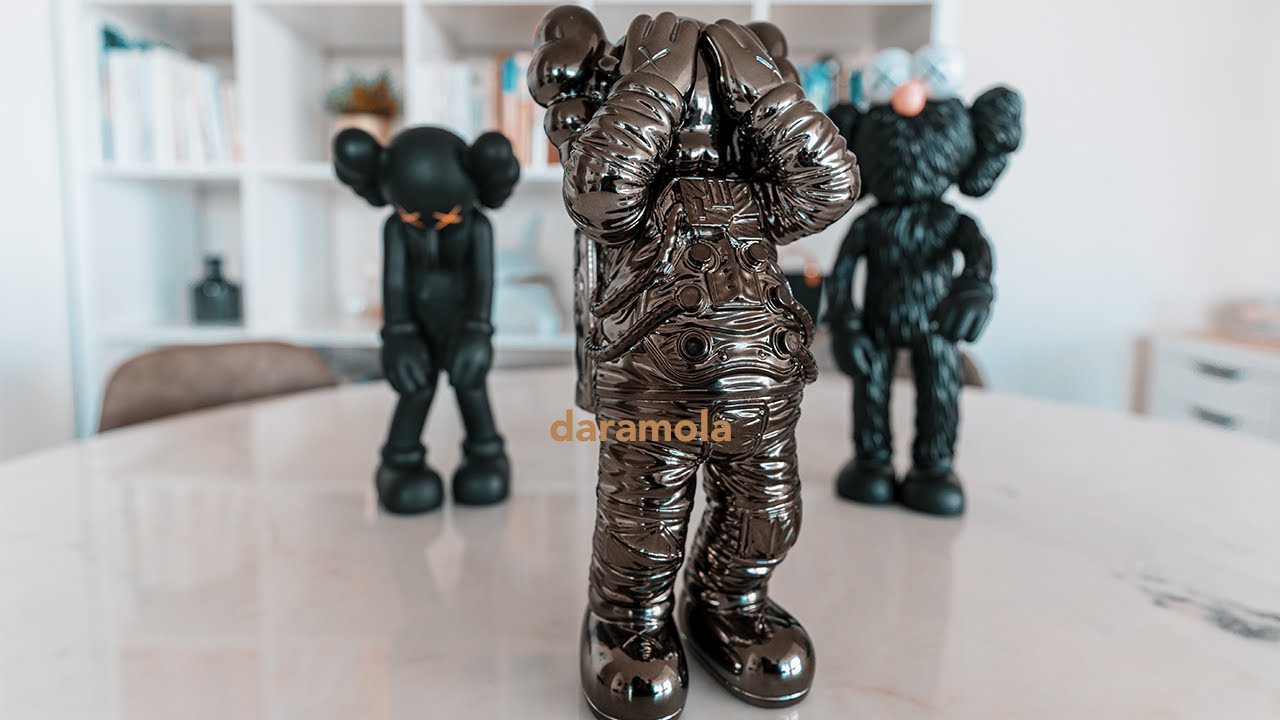In this indoor photograph, the central focus is on a detailed steel astronaut figurine, adorned in a classic spacesuit, covering its eyes contemplatively as if in a moment of despair or surprise. This astronaut figurine, placed on a tan marble table, bears the text "Daramola" at the top in a distinctive brownish hue. Flanking this centerpiece are two smaller black figurines positioned slightly behind; these figurines resemble human-like characters with pigtails reminiscent of Princess Leia from Star Wars. One has white eyes and the other has orange eyes, with one crouched down while the other stands upright. The scene is set against a blurred background, revealing part of a bookcase filled with various books and decorations to the left, and a slightly obscured set of drawers to the right.